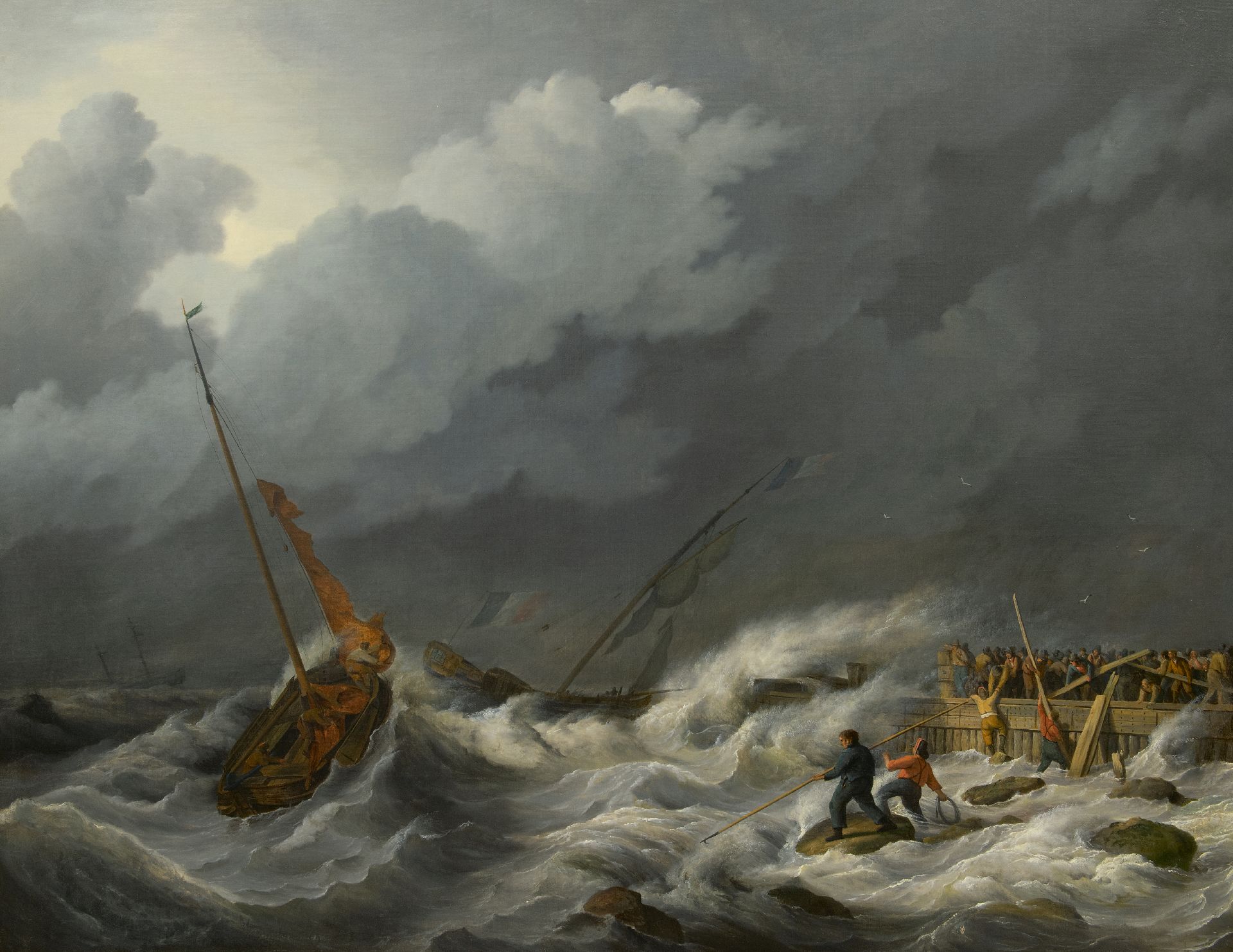The painting, likely an oil on canvas, vividly captures a dramatic and tumultuous scene at sea. The sky overhead is heavy and ominous with shades of gray and black, suggesting an impending storm. In the foreground, a small sailboat is precariously tilted, battling the fierce, crashing waves of an unforgiving sea. The boat appears to be struggling amidst the chaos, with a lone figure aboard desperately trying to navigate the harsh conditions. To the right, a larger boat is anchored near a wooden platform crowded with onlookers, their expressions filled with concern and anticipation. This platform is fenced, almost as if it provides a stage for the unfolding peril. Nearby, on a cluster of jagged rocks, two individuals stand as part of a possible rescue team—one clutching a long pole and the other gripping a rope, ready to offer aid. In the far background, barely discernible through the stormy haze, two more ships are visible, adding depth to the chaotic seascape. This powerful image encapsulates the drama of human endeavor against nature’s relentless fury.